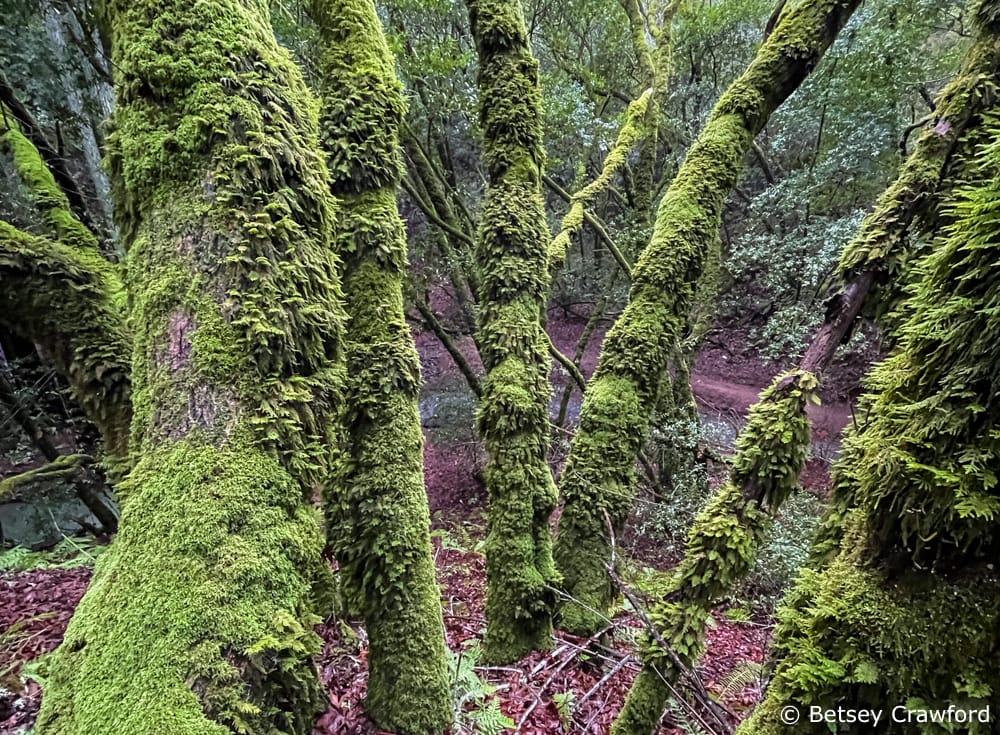The photograph captures an old, dense forest with a thick canopy of trees both upright and bent, possibly shaped by strong winds or a past tornado. The trees are cloaked in a rich, luxuriant green moss that thrives in the shady understory, extending from the base to the top of the trunks. The forest floor is layered with fallen branches and dead leaves, creating a textured, natural carpet. In the center of the image, a narrow, greenish stream meanders through the scene, adding a tranquil element to the dense woodland. The background teems with more trunks and verdant leaves, illustrating a diverse ecosystem with various tree species coexisting. In the bottom right corner, the photograph is marked with a small white copyright symbol and the name Betsy Crawford.